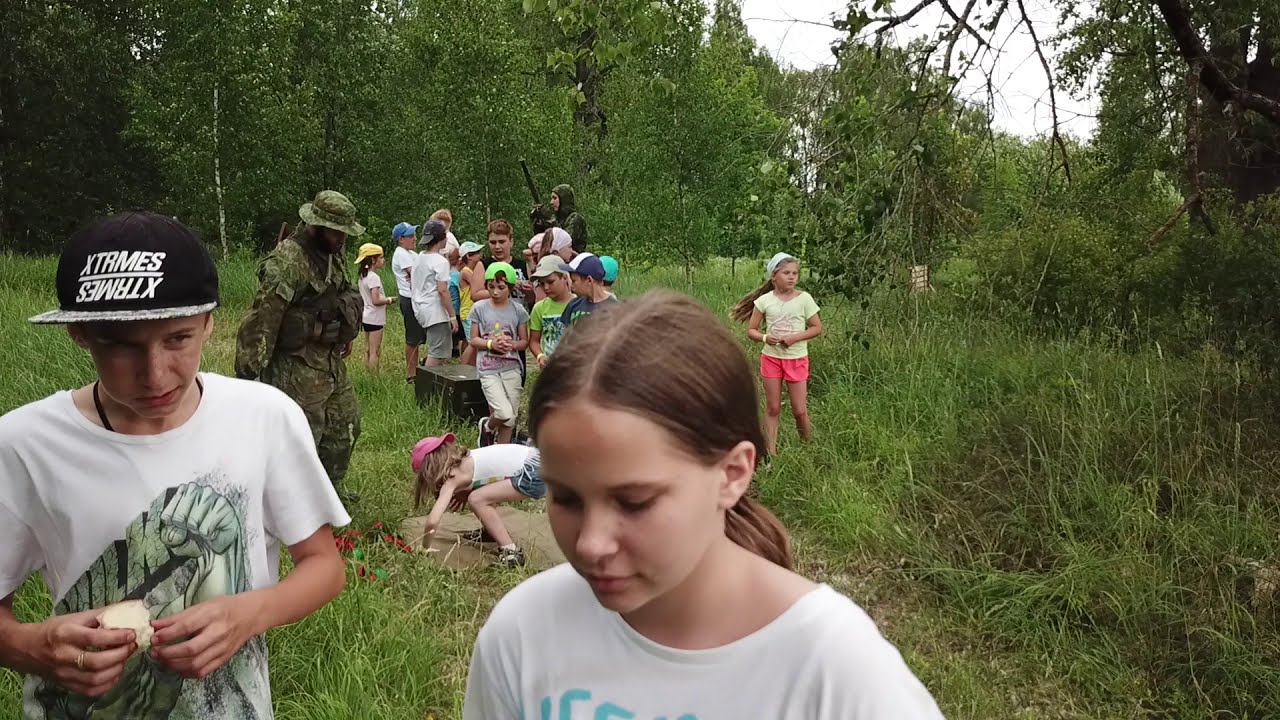The image is set in a grassy meadow with tall weeds and dense trees in the background, giving a forested appearance. In the foreground, there's a girl with long, dirty blonde hair pulled back into a ponytail. She is wearing a white shirt with blue lettering that is partially obscured, and she's looking down. Next to her, to the left, is a boy wearing a black baseball cap that reads "X-T-R-M-E-S" with a reversed version of the text beneath it. He appears to be eating an apple, with his mouth full as he glances towards the girl.

In the middle ground, there are approximately 10 to 15 children of varying ages, most of whom are wearing colorful baseball caps and t-shirts in hues of white, black, green, yellow, and blue. One notable child is a girl in red shorts. Another girl, wearing a pink hat backwards, is bending down and focused on something on the ground. She is dressed in a white tank top and blue jean shorts. Another child, a girl in pink shorts and a yellow t-shirt, stands looking at the grass with a white scarf on her head.

Flanking the group are two men in full camouflage army fatigues. One soldier, partially visible in the background, is holding a large gun. The other soldier, positioned in the middle of the children, has a beard and a hat, and appears to be observing the girl who's bending down. The arrangement suggests the children are engaged in some outdoor activity or exploration, unified by the curious presence of the soldiers amidst them.